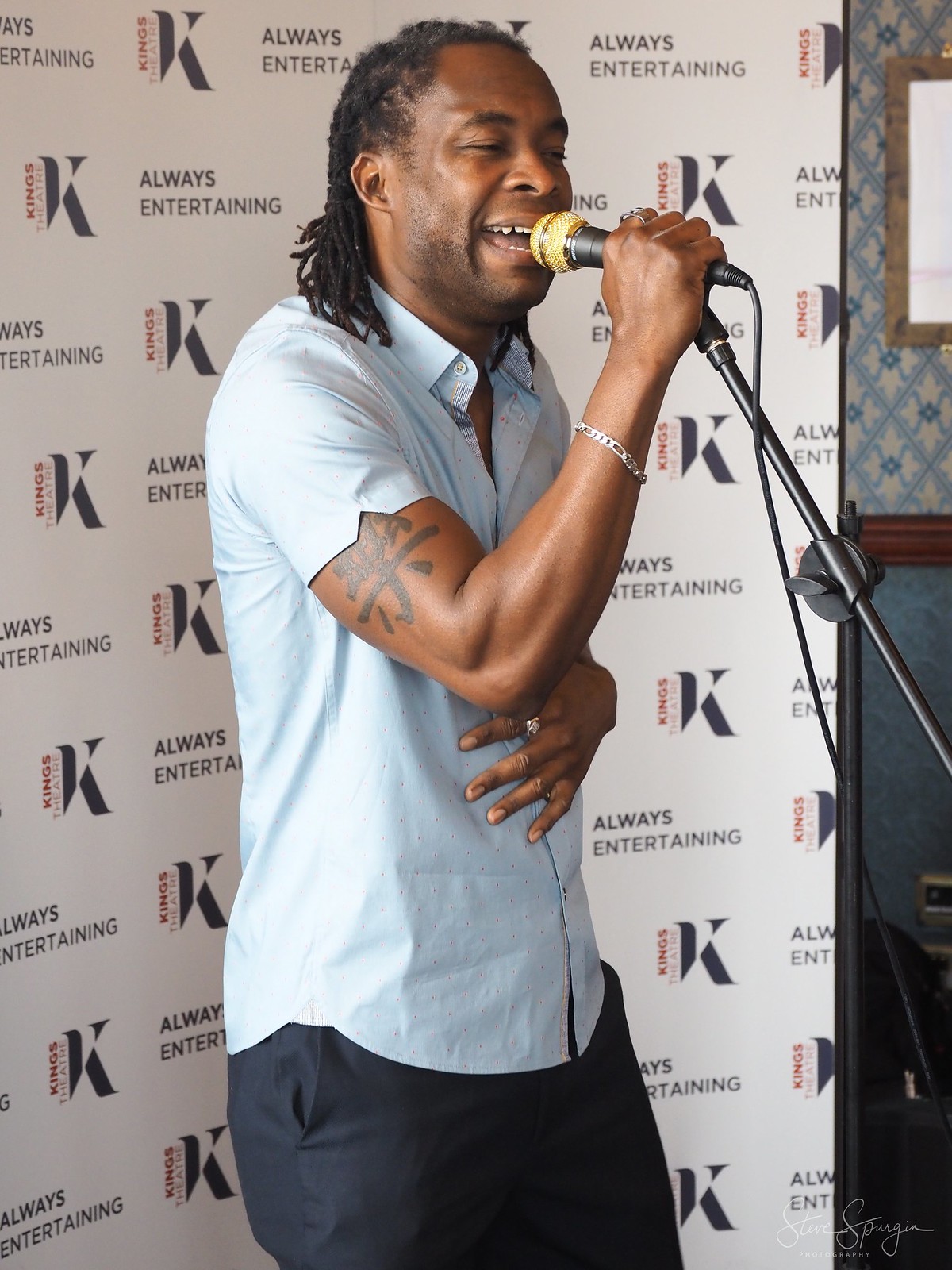The image depicts a young black man with dark, shoulder-length braided hair, mid-performance. He is singing into a gold-grilled black microphone held in his right hand, which is mounted on a tilted stand directed towards him. His light blue, short-sleeved, button-up collared shirt is complemented by dark, possibly navy blue or slate gray pants. He accessorizes with a silver bracelet on his left wrist and bears a tattoo of an oriental or Japanese symbol in black ink on his right upper arm. The backdrop features a tall white banner repeating the phrases "Always Entertaining" and "King's Theater," along with a large navy blue graphic of a 'K'. The man’s left hand is placed over his chest, highlighting his emotional engagement in the performance.